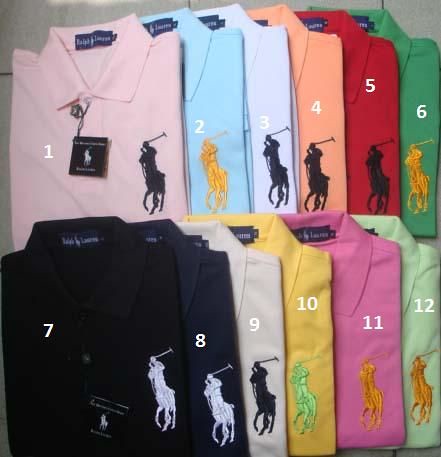This image showcases a collection of 12 neatly folded Ralph Lauren polo shirts, arranged in two rows of six against a light gray wooden background. Each shirt is distinctly numbered from 1 to 12 and comes in various colors including pale pink, light blue, lighter blue, salmon, red, dark green, black, navy blue, gray, yellow, dark pink, and light green. The polo shirts all feature the classic embroidered logo of a polo player on a horse on the left-hand breast. The tags are still visible on the front, indicating that the shirts are brand new, resembling a display one might find in a stylish golf shop or an online marketplace.